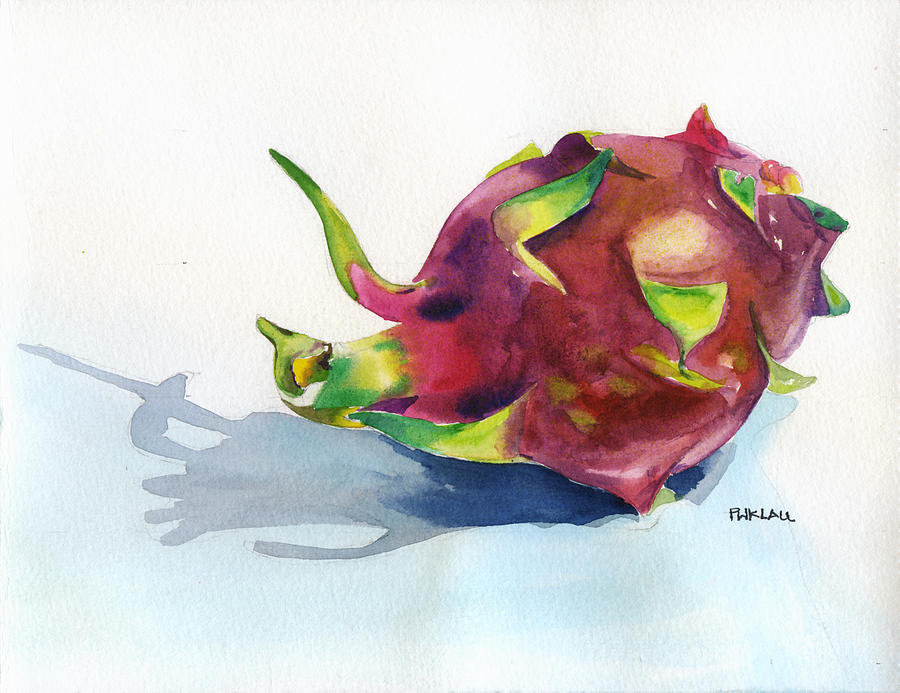This rectangular watercolor painting, which is wider than it is tall, captures a detailed and accurate depiction of a dragonfruit, though there is some ambiguity in its identification. The artwork features a dragonfruit-like shape, primarily characterized by its bright reddish-purple skin adorned with green and yellow petals or leaves extending from its body. These leaves, reminiscent of artichoke leaves, are slightly bent, adding a touch of realism to the piece. The dragonfruit is positioned slightly to the right of the center, with the stem pointing leftward. The fruit casts a shadow beneath it, painted in shades of gray and dark blue, suggesting it is resting on a light blue surface. The background remains off-white, resembling natural paper. The artwork is signed "PWK LALL" in small, uppercase black letters at the bottom right corner.